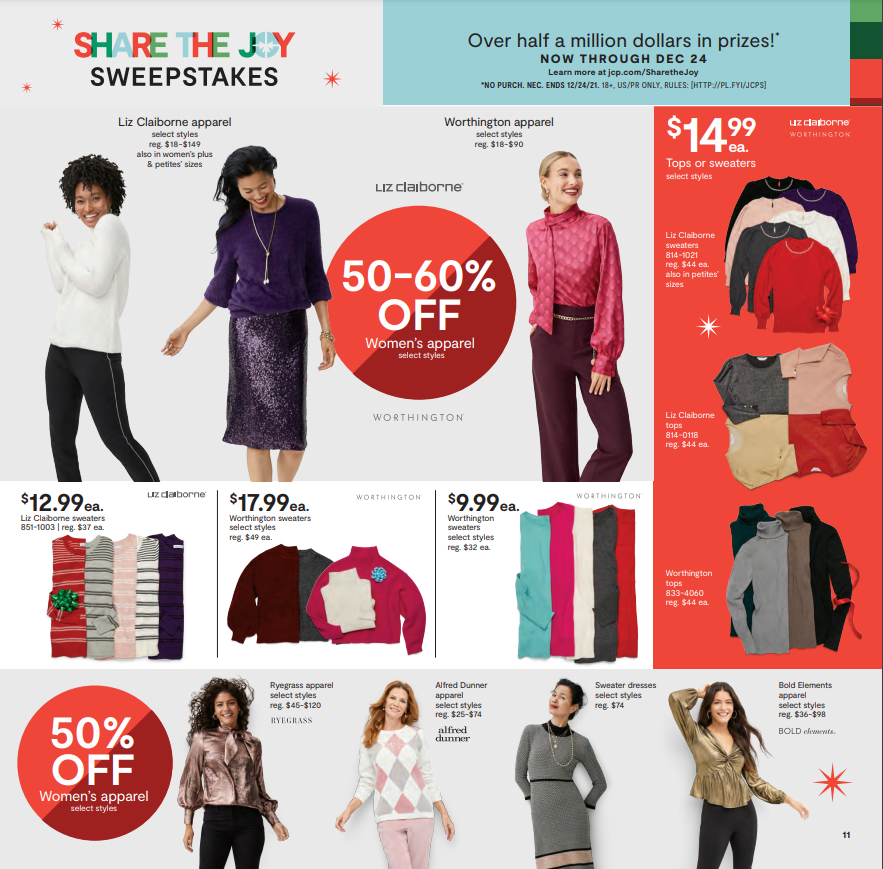The image is an advertisement poster for a clothing sale, showcasing a vibrant array of colors with red and pink as the dominant hues, complemented by accents of green, blue, white, and off-white tones, some with hints of brown and red. The top of the poster features the headline "Share the Joy Sweepstakes," with a note to the right announcing "Over Half a Million Dollars in Prizes Now Through December 24. Learn more at JCP.com/sharethejoy." Below this, there are disclaimers and additional information about the sweepstakes.

Central to the poster is a holiday sale promotion, highlighted by a large, red button stating "50% to 60% Off Women's Apparel, Select Styles - Worthington." Adjacent to this is a red banner showing various tops and sweaters priced at $14.99 each, with images and descriptions of the garments. Other sections feature more clothing items with prices listed at $12.99, $17.99, and $9.99 each, as well as another prominent "50% Off" label.

A key section of the poster displays three women modeling different outfits, each labeled with the clothing brand and the discount information. Towards the bottom, the text re-emphasizes "50% Off Women's Apparel, Select Styles," accompanied by images of four additional outfits modeled by women, emphasizing the variety and the substantial discounts available.